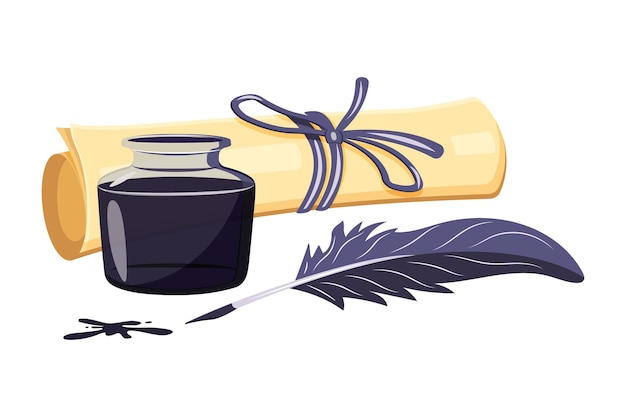This image is a cartoon drawing with a completely white background, resembling clip art and possibly created using a computer or AI. Central to the image is a rolled brown parchment, secured with a blue ribbon tied in a neat bow. In the foreground, there is a quill pen featuring a gray feather with a black-tipped nib, which has been dipped in an adjacent ink bottle filled with black ink. Near the quill, on the bottom left, there is a noticeable splotch of black ink. The dominant colors in this stylized and non-realistic illustration include various shades of gray, white, black, and blue.